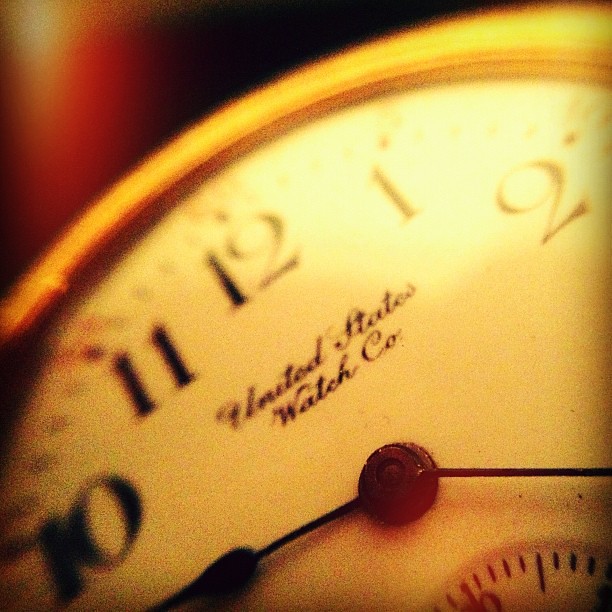This is a highly zoomed-in photograph of a watch, and the colors appear blown out, contributing to an overall brightness that obscures some details. The image exhibits a fuzzy quality, making it appear unclear. The focus is on the upper section of the watch, prominently displaying the white watch face which reads "United States Watch Company" in black cursive lettering beneath the 12 o'clock position. Only the numerals 10, 11, 12, 1, and 2 are visible, marked with dark squares and minute slashes. The hands, thin and black, are largely cropped out by the image, but the small hand is pointing to where 9 would be. A smaller dial with multiple etchings is also partially visible at the center of the watch. The watch rim has a golden or yellowish tint, and the upper left-hand corner shows a reddish glow transitioning into black, although the details are indistinct. The watch face is illuminated between the 12 and 2 positions with a bright spot, enhancing the golden-yellow hues and contrasting with the darker background.